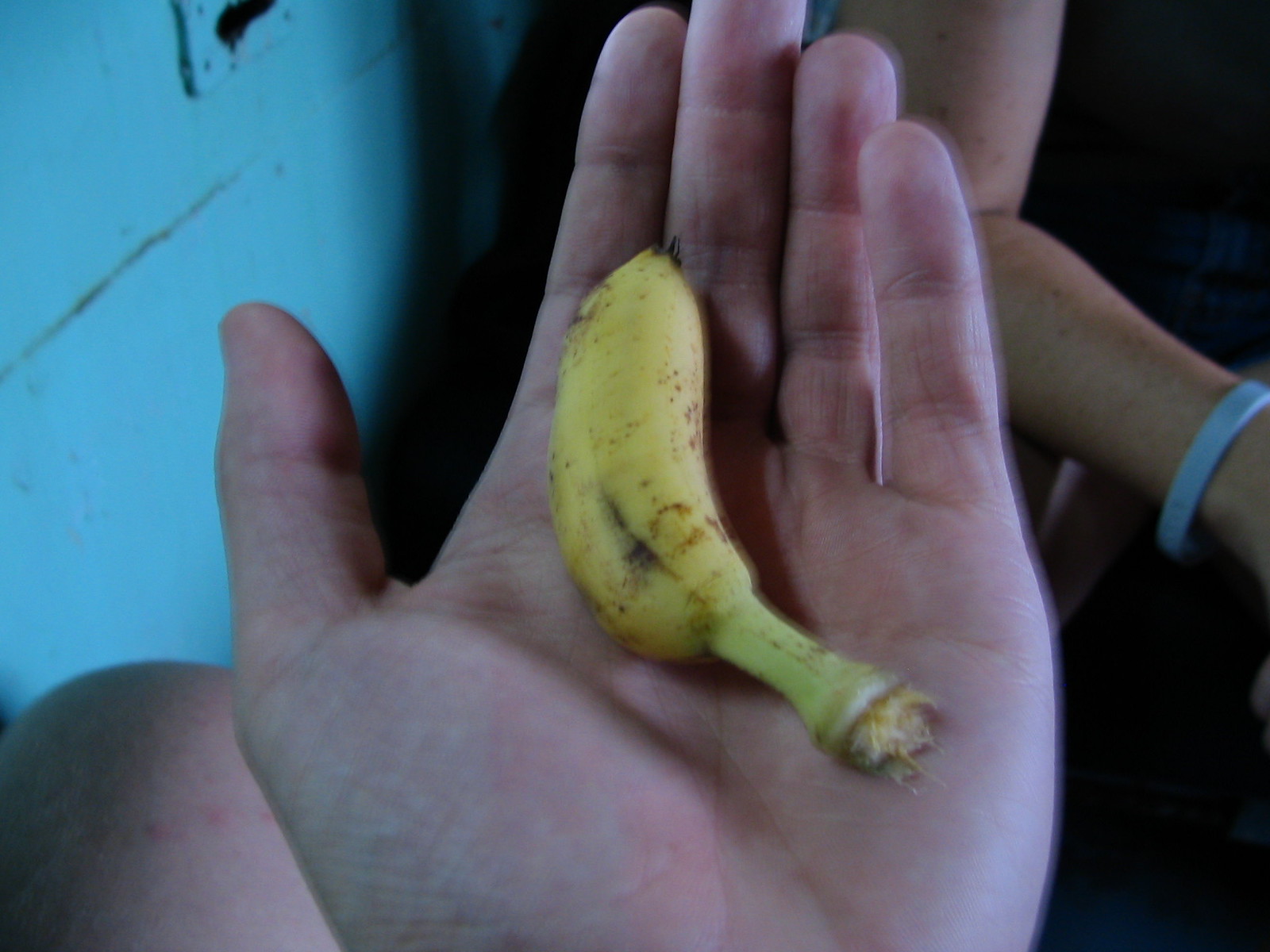The image features a close-up of a right hand's palm, holding a singular ripe banana. The hand is facing upward, presenting the banana prominently. The banana, still attached to its stem, appears very yellow with numerous dark marks and blotches, indicating its ripeness and the necessity for immediate consumption. In the background, a blue wall, marked with dark scratches and shadows, serves as a contrasting backdrop. Additionally, there is another hand visible, adorned with a light blue bangle or bracelet. The overall scene is accentuated by areas of deep shadow, adding a dramatic touch to the composition.